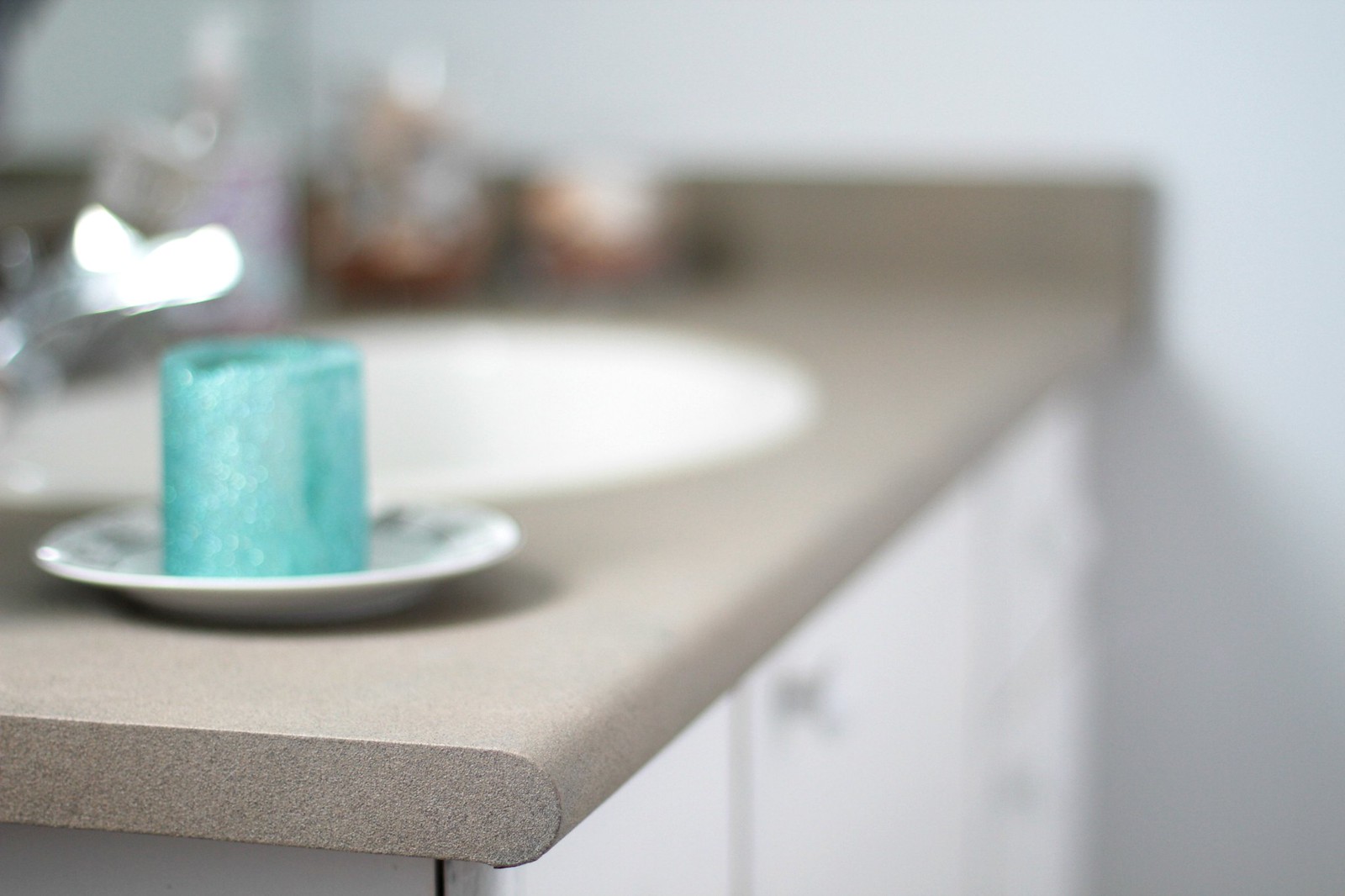The image, taken indoors in landscape mode, captures a bathroom sink and vanity from a side perspective. The photo is in soft focus, making most of the scene appear blurry. The vanity features a light gray-brown countertop with a smoothly cut, straight edge closest to the viewer. Below the counter, white cabinets provide storage. On the countertop, positioned nearest to the viewer, there is a white saucer holding a short, squat turquoise candle at its center. Just behind this setup lies a pristine white sink paired with a sleek chrome faucet. In the back corner of the sink area, a series of glass jars of graduating sizes can be observed, although they remain out of focus. The only part of the image in clear focus is the edge of the countertop closest to the viewer, showcasing its sharp, well-defined cut.